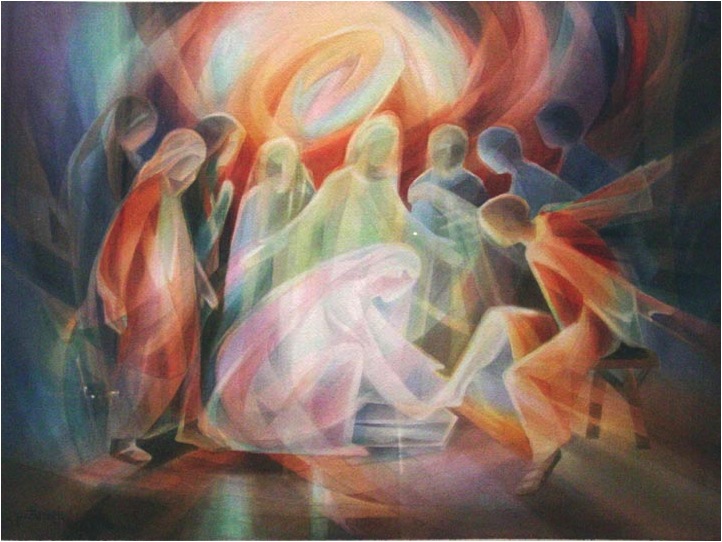The artwork is a painting depicting a ghostly, ethereal scene with a central, kneeling figure who might be reminiscent of Jesus. This figure, bathed in a ghostly white hue, is touching the foot of a seated person to their right, who is dressed in an orange robe and appears to be somewhat unbalanced, reaching back as if to steady themselves. This seated person's foot is also turning white where it contacts the kneeling figure, suggesting a transformative or cleansing act akin to a foot washing. 

The background is a mesmerizing swirl of multicolored, almost translucent paint, contributing to a three-dimensional effect. This kaleidoscopic backdrop, blending red, yellow, green, and blue, enhances the surreal and spiritual atmosphere, appearing almost like a portal. Surrounding the central figures are about eleven human-like individuals, distinguishable by their vivid, solid-colored tunics and scarves—green, blue, red, and other hues—yet they have blank, faceless heads. They seem to be spectators, encircling the scene with one figure in the center extending its arms outward, drawing attention to the miraculous event before them.

The overall composition evokes a dynamic, ghostly assembly immersed in an otherworldly ambiance, with its swirling colors and crowd of onlookers emphasizing the significance of the central act.